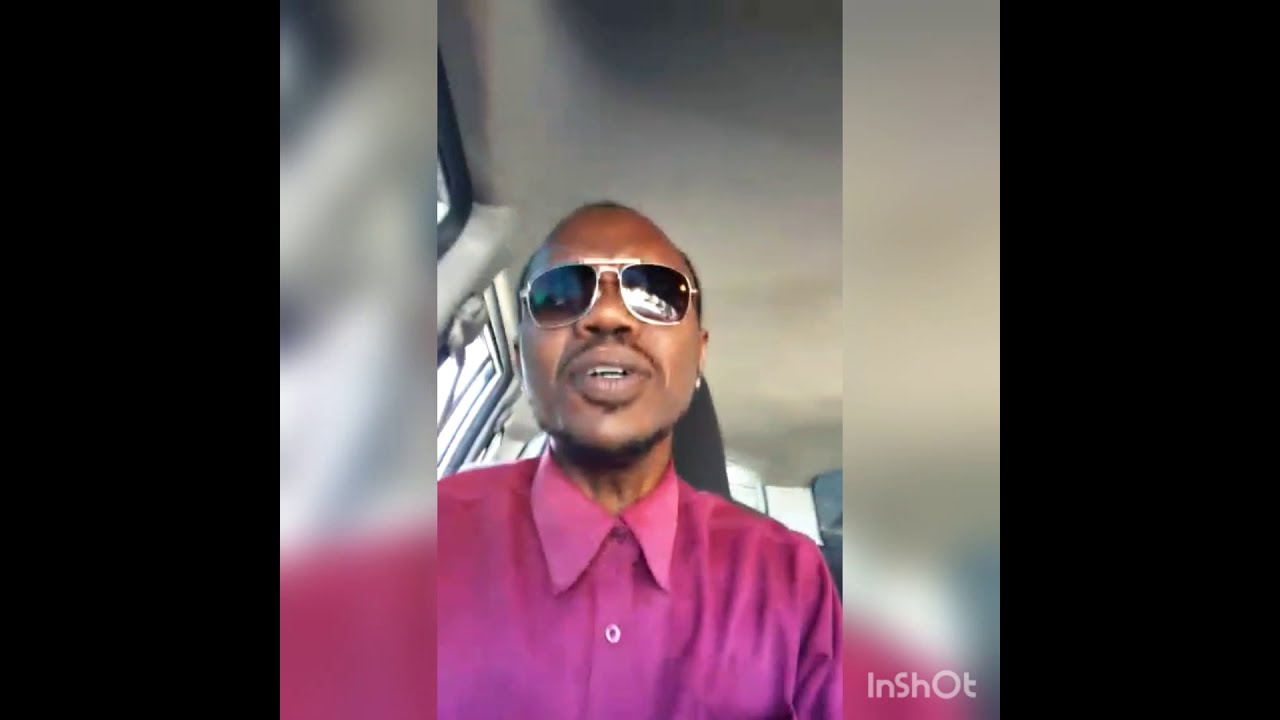The image features a vertically-oriented selfie or screen grab from a selfie video of an African American man, likely captured from a cell phone. He is in the interior of a vehicle, possibly a car or van, distinguished by its grey roof and windows. The man is bald or balding, has facial hair on his chin and neck, and is wearing dark sunglasses with gold rims. He is dressed in a buttoned-up dark pink shirt. The camera is positioned below his face, looking up at him, and he appears to be speaking into the camera. 

The image itself is divided into three panels: a large central panel and two smaller, blurry, out-of-focus panels on either side that are zoomed-in sections of the main image, specifically his left and right shoulders. These panels are flanked by black bars, adding to the vertical cell phone image's wide rectangular appearance. Additionally, there is a watermark "InShot" at the lower right corner of the image, indicating the use of a video editing app.